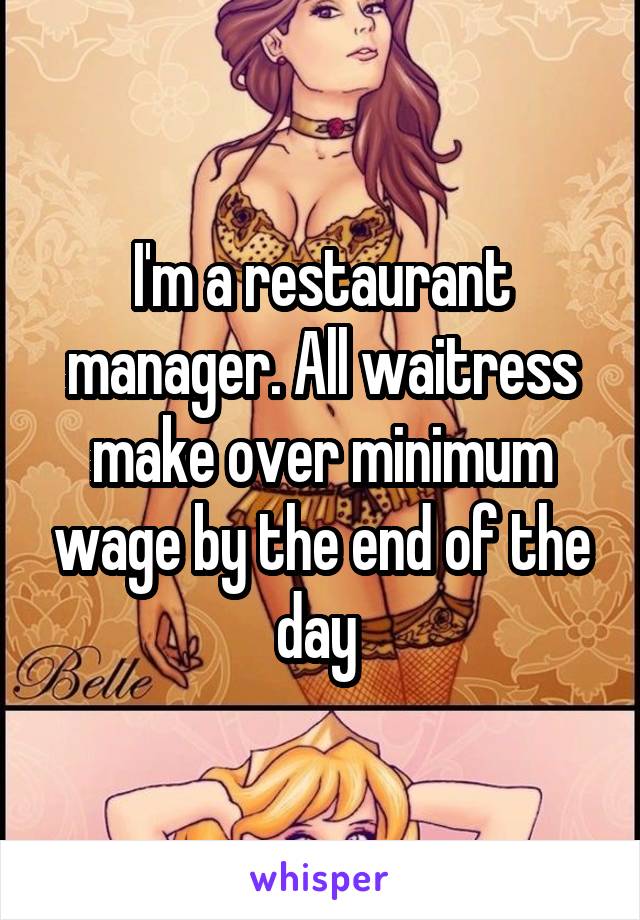This image features a detailed cartoon drawing in a fantasy anime style of a Caucasian woman with long, wavy brownish-reddish hair, standing provocatively in yellow lingerie, including a bra and very short skirt, accompanied by fishnet stockings and a choker necklace. She gazes directly at the viewer with a seductive expression. Above her head, text reads: “I am a restaurant manager, all waitresses make over minimum wage by the end of the day.” The backdrop is elaborately decorated with cream and goldish-tan floral and leaf patterns, giving it a luxurious feel. In the bottom left corner of the image, the word “Belle” appears, presumably the woman's name, written in black. Below this main depiction, the top of another cartoon image can be seen, showing just the head and hands of a blonde woman with her arms lifted overhead. Below this partial image, the word “Whisper” is written in purple against a white background. The overall scene suggests some form of advertisement or promotional material.